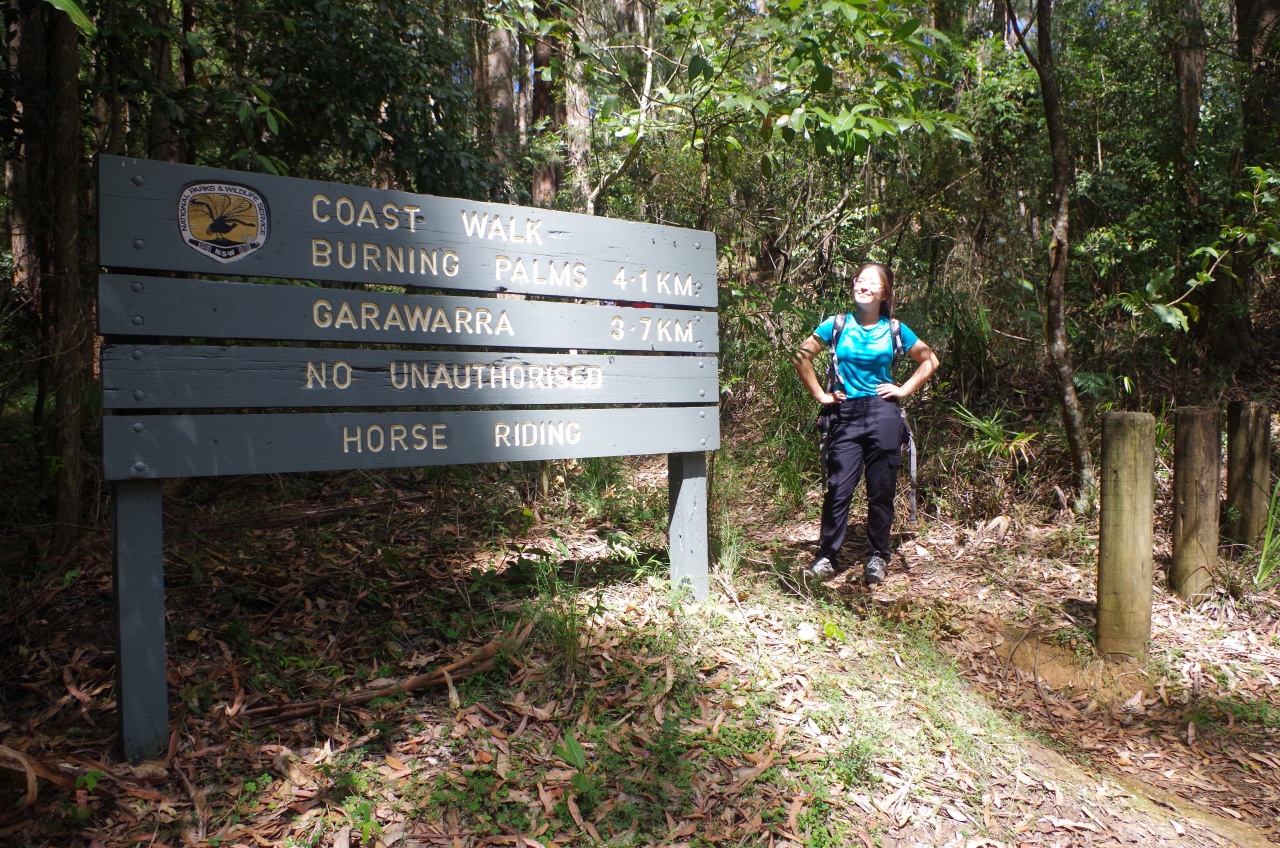The image captures a young woman, possibly of Asian descent, standing outdoors in a forested area during daytime, with the sun shining brightly. She is wearing a teal blue shirt with a print on it, black pants, hiking shoes, and a backpack, indicated by the straps over her shoulders. Her brown hair frames her face, which is adorned with glasses and a cheerful smile, suggesting that she is enjoying her time outside.

She stands on a dirt and rocky path, surrounded by tall trees and grass, with leaves scattered on the ground. Crowning the scene is a four-slatted wooden sign held up by two posts. The black and white sign reads: "Coast Walk, Burning Palms, 4.1 kilometers," followed by "Garawara, 3.7 kilometers," and finally, "No Unauthorized Horse Riding." Additionally, to her left are three visible round cement poles about three feet tall.

Her stance, with both hands on her waist, shows she is absorbed in reading the sign, perhaps planning her next move on the hiking trail.